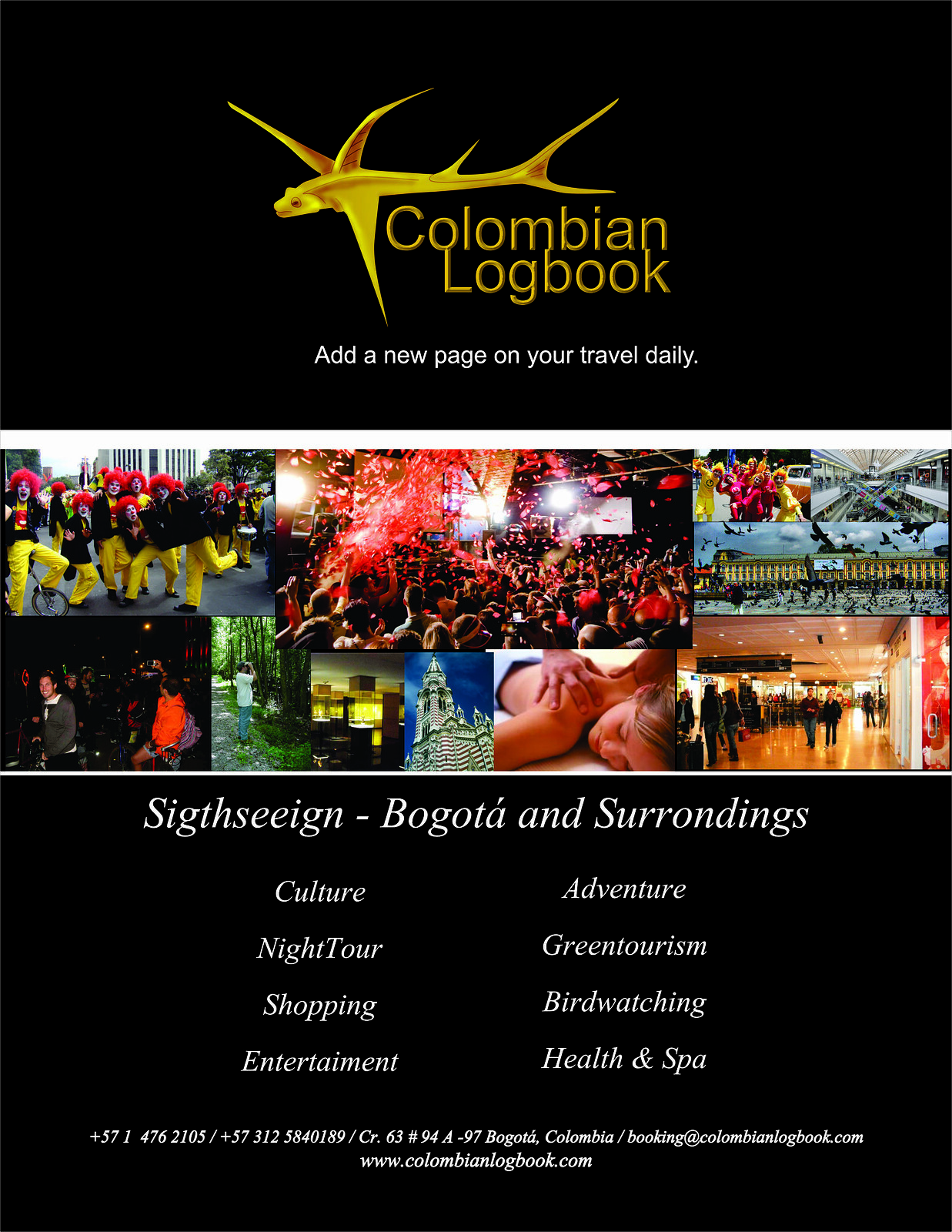This advertisement poster for travel to Colombia features a striking design set against a black background. Dominating the top is a distinctive golden logo depicting a stylized flying fish with six fins—two side fins, three dorsal fins, and one bottom fin that extends to the back tail. Below the logo, in elegant golden text, is the name "Colombian Logbook" followed by the enticing slogan, "Add a new page to your travel diary," rendered in white.

At the center of the poster is a vibrant collage of approximately eight photographs, capturing the diverse activities and attractions Colombia offers. The images depict a lively carnival scene with confetti, people dancing at what appears to be a dance club, an individual enjoying a soothing back massage, shoppers in a bustling mall, an outdoor concert, nature enthusiasts amidst lush greenery, and clowns bringing joy to spectators. The vivid colors in these photos range from red, blue, and green to yellow, orange, and more, providing a kaleidoscope of experiences.

Beneath the collage, detailed in white text, are the highlights of what travelers can expect: "Sightseeing, Bogota and surroundings, Culture, Adventure, Night tour, Green tourism, Shopping, Bird watching, Entertainment, Health and Spa." At the bottom of the poster is the website address, www.colombianlogbook.com, inviting viewers to explore further.